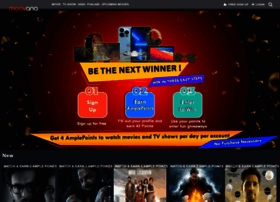The image depicts a promotional advertisement for a website or app that appears to be named "Muvana" or "Munana," though the exact name isn't entirely clear. The design suggests that it is a streaming platform specializing in TV shows and movies. Central to the ad is the slogan "Be the Next Winner," displayed prominently on a yellow flag-like banner with black text. This tagline hints at an ongoing contest, presumably offering various prizes.

The promotional materials showcase potential prizes, including a smartphone, headphones, and what could be a computer monitor or desktop setup. A "Sign Up" button is visible alongside two additional call-to-action buttons in blue and aquamarine, although the text on these secondary buttons is not legible.

The advertisement briefly mentions a daily offer of "four in web movies and TV shows," though this text is partially obscured. Below this, five TV show thumbnails are displayed, all featuring characters with brown skin tones, indicative of Indian origin:

1. The first thumbnail on the bottom left features a man wearing black-rimmed glasses.
2. The adjacent thumbnail shows a bearded man holding another person who appears to be injured.
3. The middle thumbnail is indistinguishable.
4. The fourth thumbnail seemingly depicts a scene from a superhero film, with a bearded man conjuring flames.
5. The fifth and final thumbnail shows a man with brown hair and a goatee, set against a cloudy backdrop.

The lack of specific show titles suggests these are new releases exclusive to the platform. The overall aesthetic and content imply that this streaming service is tailored to an Indian audience, offering a range of new TV shows and movies.